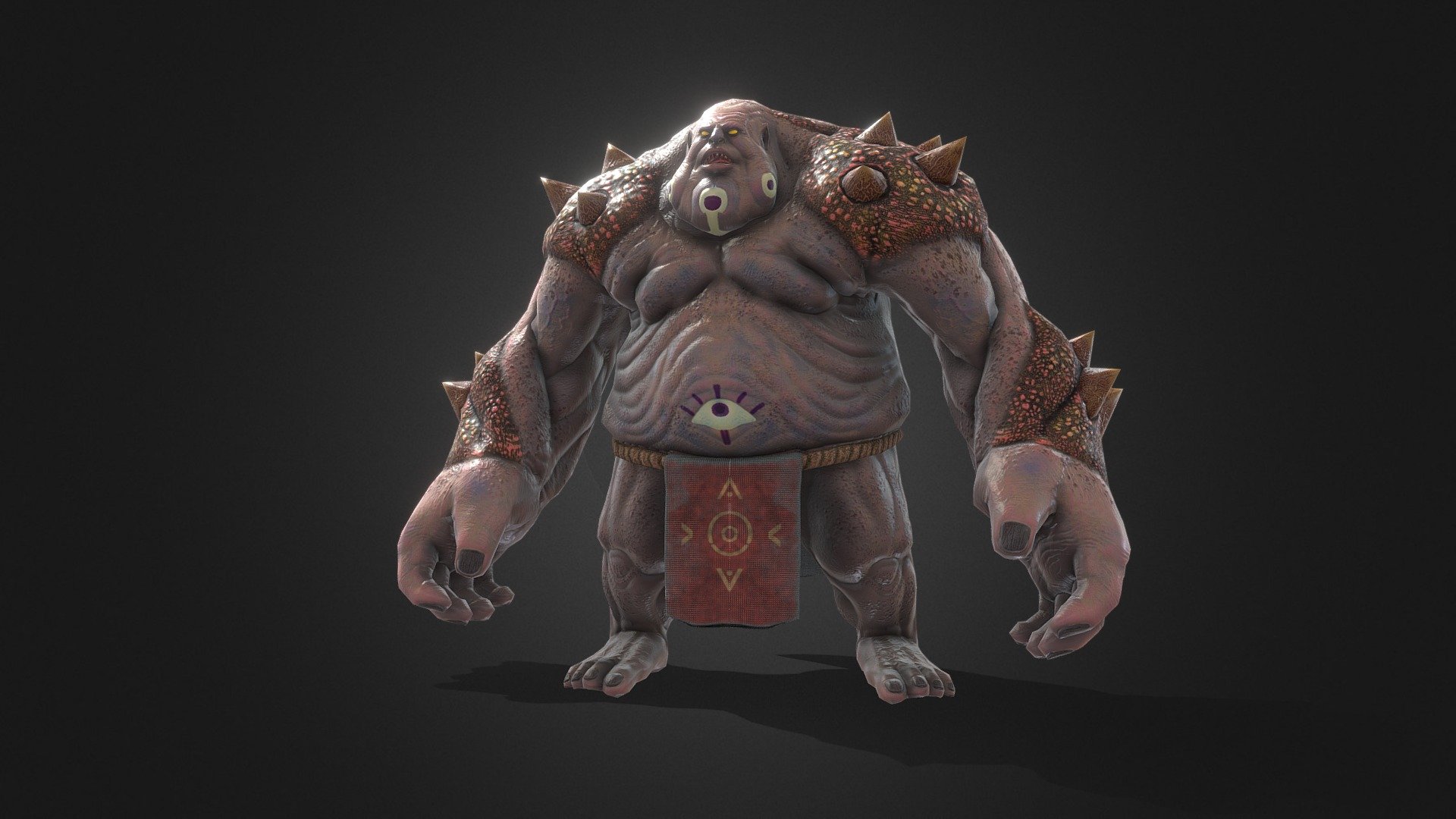The image depicts a large, fantastical creature that resembles a monstrous troll or beast. Its skin is dark gray with a purplish hue, appearing scaly in texture. The creature has a very elongated, oval-shaped face, marked with a prominent chin adorned with a white strip down the center and a black dot just below its mouth. Its mouth is open in a frown, and the jaw area features face paint.

The creature's imposing physique includes an oversized torso and remarkably muscular arms that nearly reach the ground, ending in enormous hands with dark fingernails. It wears grand shoulder pads colored in shades of brown and yellowish tones, adorned with large, protruding spikes. Matching spiked wristbands accentuate its forearms.

The chest of the creature is somewhat irregular, with small pectoral muscles and a rounded, protruding belly. An eye-like design, complete with eyelashes and a black dot in the center, decorates the belly button area. From its waist hangs a thin gold belt, and covering its pelvic region is a red cloth featuring intricate gold and red patterns. This design includes concentric circles and the letter "A" shapes positioned both upright and upside down, flanked by inward-pointing "V" shapes.

The creature's short yet heavily muscled legs end in large, barefoot feet positioned towards the camera, casting a shadow underneath that extends to the bottom right corner of the image. The background transitions from a black outer edge to a lighter gray surrounding the creature, highlighting its ominous and fierce presence.